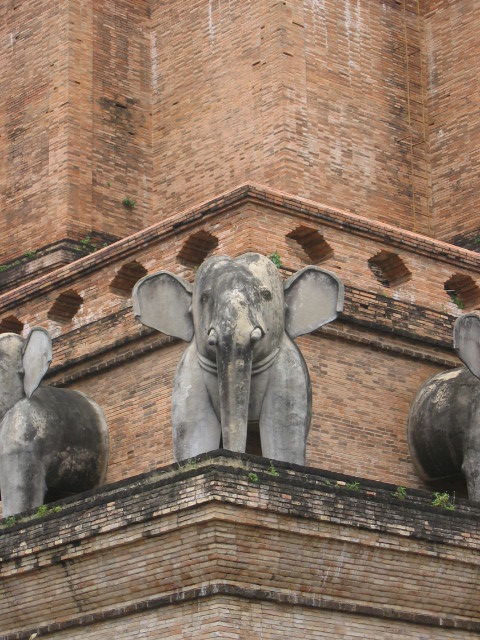This photograph captures the weathered charm of an aged brick building featuring a trio of elephant statues that adorn its corner. The building is constructed from a variety of brown and tan bricks, showing signs of aging and decay, with patches of dirt and varied colors adding to its historic allure. The primary focus of the image is a close-up of one central light gray elephant statue, positioned prominently at the corner, facing forward with its tusks pointing directly at the viewer. This main statue exhibits a mottled appearance, with darker gray patches speckling its trunk and ears. Flanking this central statue, two additional elephants are partially visible, sharing the same light gray tone and detailed craftsmanship. Surrounding the statues, a solid ledge shows signs of greenery sprouting from it, and above the elephants, intricate hexagonal patterns are etched into the brickwork, adding to the architectural intricacies of this storied structure.